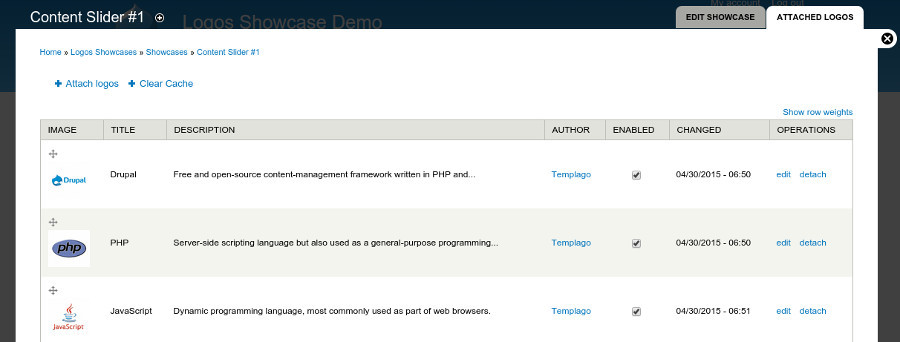This image showcases a detailed view of a website management interface on a computer screen. The page appears to be part of an administrative dashboard where businesses can manage their branding materials, such as logos and other promotional content. The interface features a navigation menu with options like "Home," "Logos," "Showcases," and lists "Content Slider Number One" as the current section.

At the top, the interface allows users to edit showcased logos. Below this, there is a chart displaying detailed information for various logos. The chart columns include "Image," "Title and Description," "Author," "Enabled Status," "Last Changes Made," and "Operations."

In the chart, there are entries for logos, such as one for "Drupal." The logo for "Drupal" is a small image, and its description starts with "This is a free and open-source content management framework written in PHP," but the text is cut off. The author for all entries is listed as "Templags." All the listed logos have the "Enabled" box ticked, indicating they are active. The last status update for these entries was made on April 30, 2015, at 6:50.